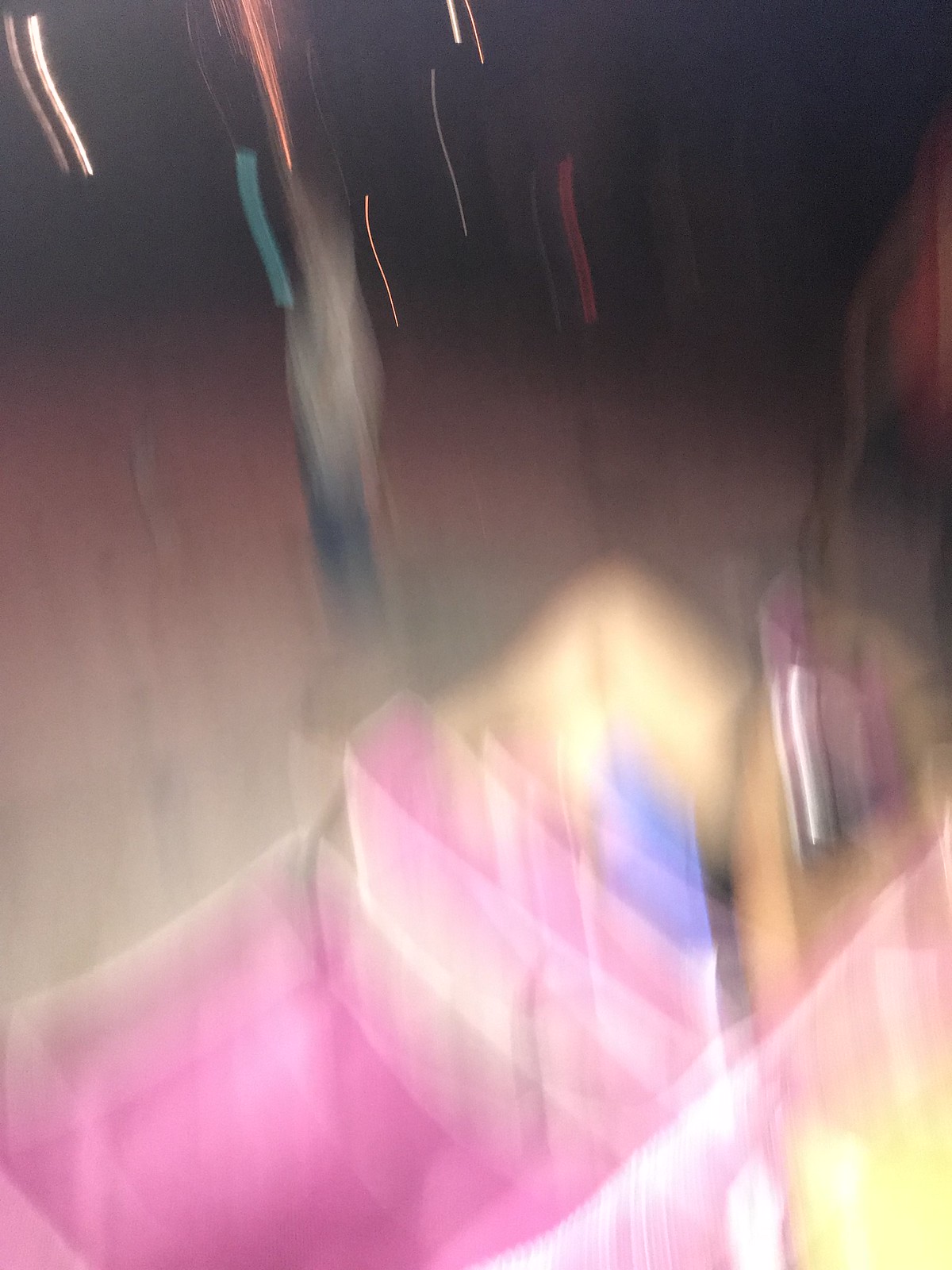The image is a highly out-of-focus, close-up photo, making it difficult to discern specific details. It appears to capture a scene at night, possibly outdoors, featuring streaks of multicolored lights — red, orange, blue, white, green, and yellow — creating a surreal, blurry effect. In the center of the image, there's a vague outline of a standing person, potentially a woman with dark hair, wearing a pink tank top and shorts, though patterns on the clothing are indiscernible. Another possible figure may be present, seemingly in blue jeans and a white shirt. The bottom right corner hints at a complex mix of objects and colors, including something resembling a pink basket with objects inside it, and nearby, a yellow element and some tan, skin-like hues, possibly indicating another part of the person's body or a different object. The entire scene exudes a sense of chaotic motion, as if the photo was taken while moving, contributing to its overall blurriness and unclarity.